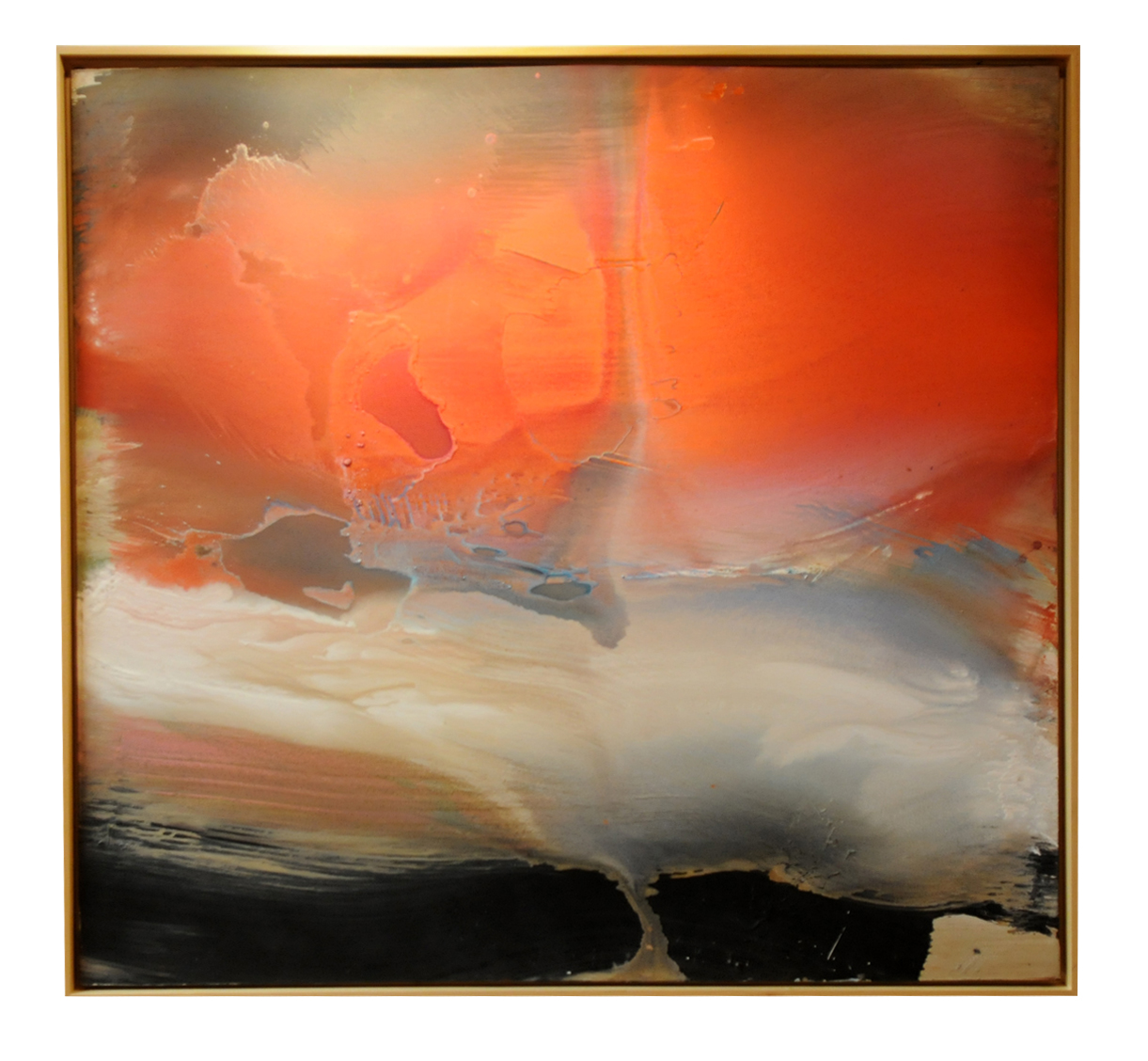The painting is a square abstract piece framed with a light brownish gold border, set against a white background. Dominating the top half of the artwork is a very bright and deep orange color that transitions into a darker orange hue towards the right side. The texture here is organic, with visible strokes and smears suggesting the use of a palette knife. Interspersed within this orange field are softer areas of beige and white.

Beneath the vibrant orange, the painting features an abstract shadowy area composed of light gray, bluish, and orange hues. This middle section creates a subtle transition between the vivid top half and the darker bottom half. 

At the bottom, a prominent black horizontal area spans across the painting, starting higher on the left, dipping down, slightly rising, and then descending towards the bottom right corner. Within this dark region, a light brownish-green form interrupts the black expanse in the center, and a similar hue appears as a splotch in the right corner. Additional patches of blue-gray and beige are visible towards the left and right sides, enhancing the complexity and depth of this painting. The abstract composition and rich texture make for a visually compelling and dynamic artwork.